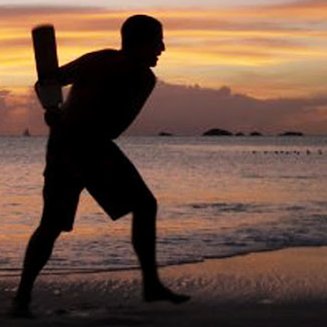At dusk on a serene beach, a silhouette of a man, poised to swing a rectangular cricket bat, stands against a breathtaking backdrop. The man, facing right, is captured mid-motion with the bat slightly behind his back and poised toward the upper left corner. He is dressed in shorts and a sleeveless shirt, his bare feet grounded in the dark, almost black sand. The left foot is turned toward the right, and his right foot points slightly toward the camera, emphasizing his stance. His silhouette is outlined starkly against the calm, bluish water, which reflects the yellow illumination from the setting sun. The expansive ocean spans halfway up the picture, with distant mountains adding depth just above the horizon. The sky transitions from dark clouds rising from the mountains to a blend of blue, with scattered white and yellow clouds. This mesmerizing image captures a moment of calm anticipation under a richly colored dusk sky.